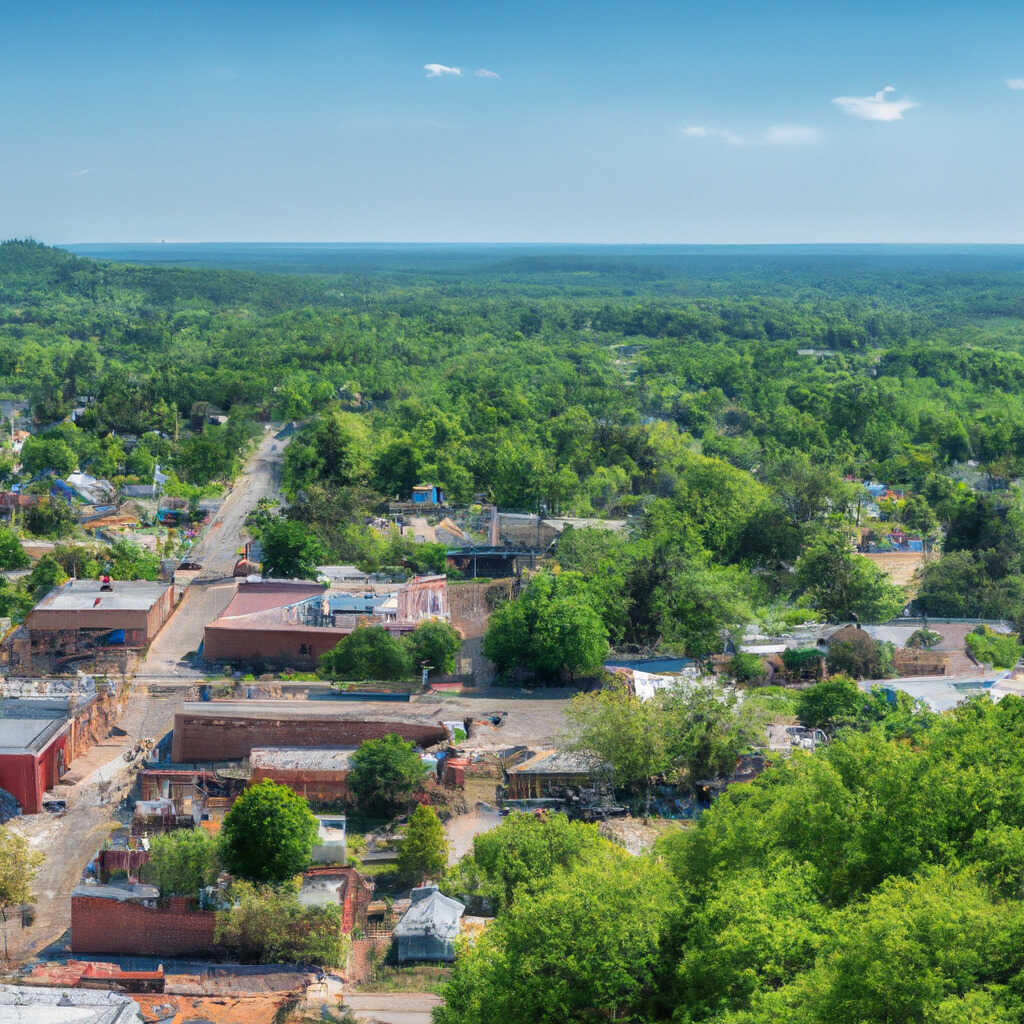This image captures a high-angle, oblique overhead view of a small village or town, likely photographed from a drone or a hilltop. The photograph, which seems to have a slight saturation hinting at an older era, is squared in shape, measuring approximately 5 to 6 inches in both height and width. From the upper third of the image, the dark blue sky transitions to a lighter bluish-gray near the horizon, dotted with a few small white clouds. Beneath this, the scene reveals a dense tapestry of greenery and forested areas interspersed with a mix of older, low-lying buildings, many of which appear to be in disrepair, implying potential impoverishment. The buildings vary in color, featuring shades of pink, red, and yellow, standing out vividly amongst the green treetops that cloak parts of the village.

Two main intersecting streets organize the layout of this town, with one street running vertically and the other horizontally. These roads are bordered by a mix of squat warehouse-type structures and residential houses, typically no more than two stories high. On the left-hand side, a wide paved road connects with several intersecting roads and is lined with more substantial, square brown buildings. An area resembling a sports court or open paved space is also visible.

Amidst the varying vegetation and buildings, the town appears devoid of cars or vehicles, and only a few people can be seen on the left-hand side, seemingly moving in the same direction. The composition raises curiosity about its reality, as the absence of vehicles and the overall scene lends an impression that it might actually be a model or painting rather than a photograph, although this remains ambiguous. The image evokes a sense of nostalgia and curiosity, blending the vibrancy of the town with the encroaching wilderness.